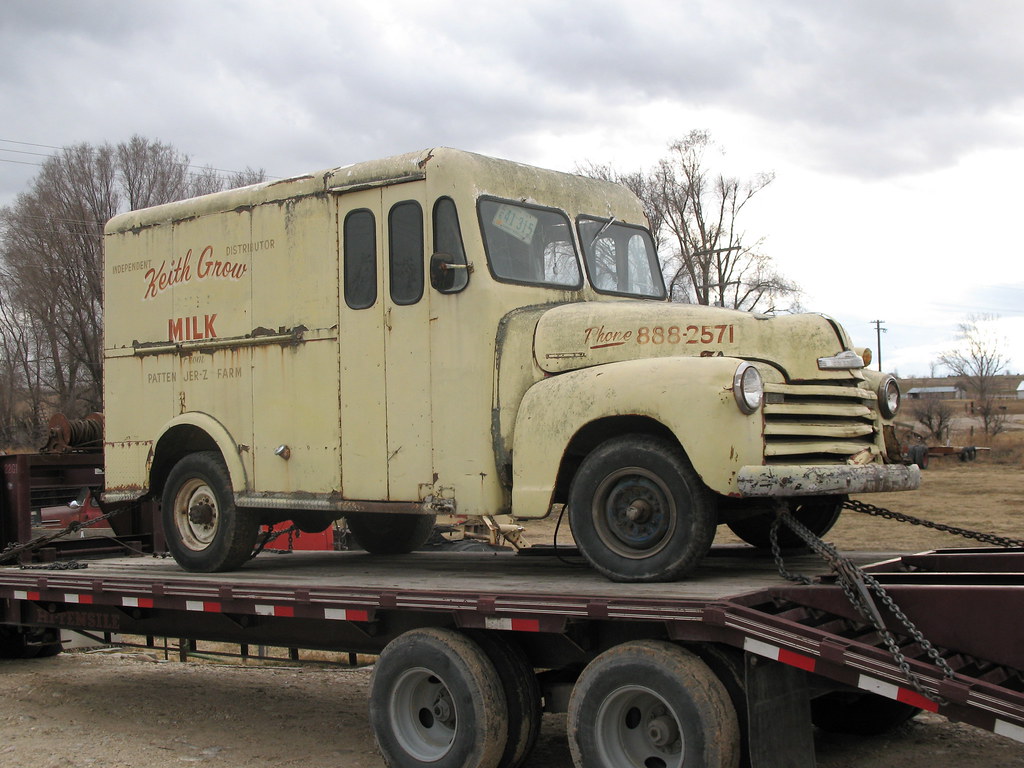The image depicts a vintage milk truck, estimated to be from the 1930s to the 1960s, secured on the back of a flatbed trailer. The truck, predominantly a dingy yellow with noticeable wear and missing hubcaps, features red cursive lettering on its side that reads "Keith Grow Milk" and "Patton Jersey Farm," identifying it as an independent distributor. There's an old phone number "888-2571" visible on the truck, likely no longer in service. The truck, with a pointed hood and horizontal metal grates on the front, has doors that open similarly to a school bus. It is fastened backwards on the trailer, which is facing left, indicating that the truck’s front is oriented to the right within the image. The outdoor setting includes a mostly gray, overcast sky with barren trees and telephone poles on the left, and some brown grass and additional trees on the far right. The truck appears neglected and possibly en route to a junkyard.